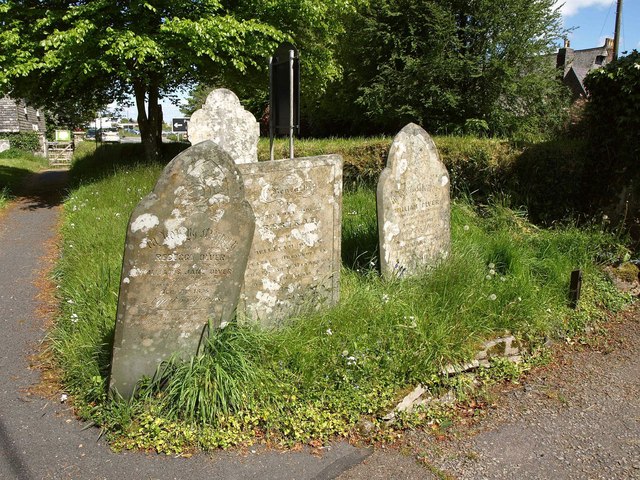The photograph captures a small, grassy plot featuring four weather-worn gravestones, each inscribed with barely legible writing in an old-fashioned font. The headstones vary in shape: two have pointed, curved tops; a rectangular one sits in between them; and a taller, lighter gray headstone with a curved but non-pointed top stands behind the three. This plot is bordered by a paved walkway, which curves from the left side of the image, passes through a gate, and stretches across the foreground. Notable elements in the background include two partially visible houses—one obscured by a large tree on the left, and another peeking from the right. Additional background details include a road with a couple of cars and some trees, contributing to the serene, slightly somber ambiance of the setting that suggests it may be part of a cemetery or a personal burial ground.